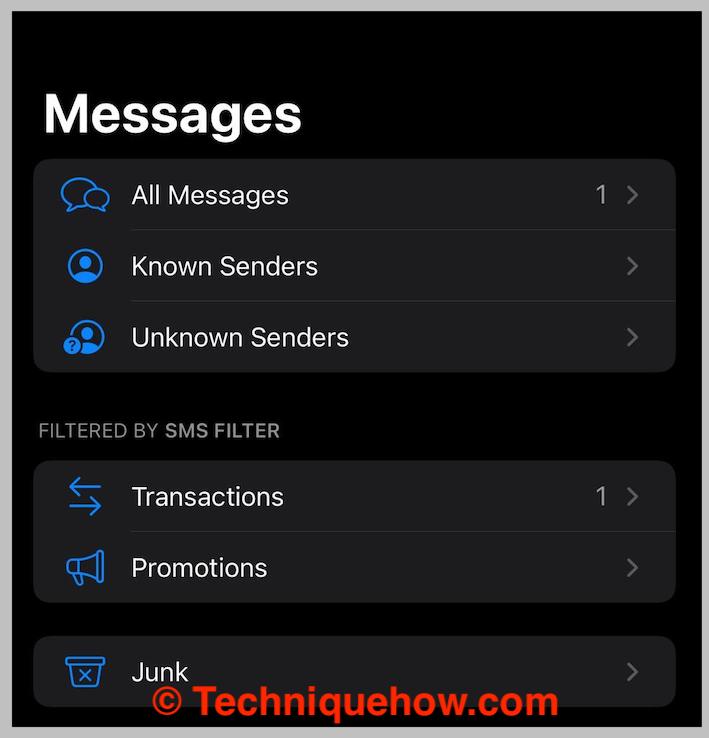The image depicts a "Messages" screen on a mobile device in dark mode. The background is black with gray sections highlighting various menu options. In the top-left corner, "Messages" is prominently displayed in bold white font. Below this title, in a gray section, there are blue icons: a thought bubble and two profile icons overlapping each other. Next to these icons, three white text labels read "All Messages," "Known Senders," and "Unknown Senders," respectively. "All Messages" has a notification badge with the number one on the opposite side.

Further down, below another gray section, it reads "Filtered by SMS Filter" with categories listed underneath: "Transactions" with a '1', and "Promotions" with no number. A megaphone icon is placed next to "Promotions." The last gray bubble contains the label "Junk" in white text, accompanied by a blue trash can icon with an X over it. At the very bottom of the screen, a red copyright notice displays the text "techniquehow.com," with each letter clearly spelled out as T-E-C-H-N-I-Q-U-E-H-O-W.com.